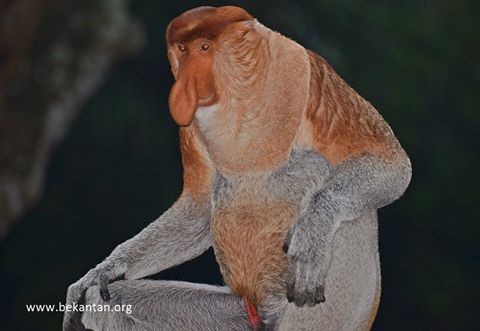In this image, we see a unique primate which appears to be a type of monkey or ape, prominently positioned towards the center, facing slightly to the left. The background is a dark green blur, likely foliage, although the details are indistinguishable. The monkey has a distinctive large, droopy orange nose and small mouth. Its beady red eyes are accentuated by the dark, indented crown on its head, with fur transitioning from dark brown to reddish-orange around the neck and shoulders. The fur is predominantly gray starting from the elbows down to its fingertips, the latter being a very dark gray or almost black. Its torso features a brownish belly transitioning to gray again at the top of its legs. Notably, one leg is extended forward while one hand rests on its knee, and the other hand hangs by its side. The image is marked with the watermark "www.bekantan.org" in white text at the lower left corner.